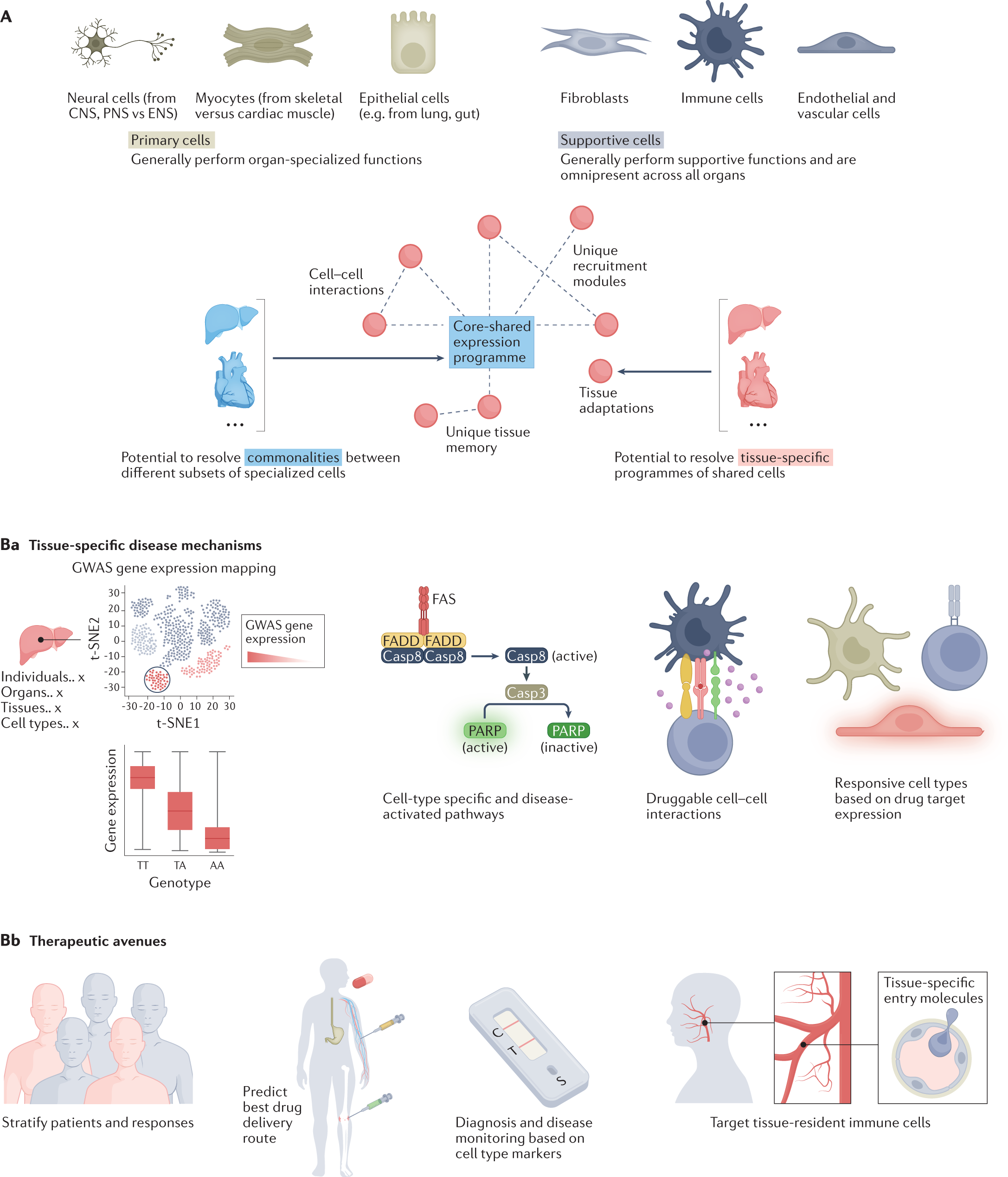This is a comprehensive and detailed medical illustration labeled ABA and BB, designed for educational or presentation purposes. The diagram showcases a multitude of cellular processes, focusing specifically on cell-cell interactions, neural cells, myocytes, immune cells, and their roles in various tissue-specific disease mechanisms and cell type-specific disease-activated pathways. The chart is richly colored with distinct hues to represent different cellular functions and mechanisms, set against a white background, with extensive black text annotations.

At the top left, there are detailed depictions of neurons and epithelial cells, with accompanying black text descriptions. Gray-colored illustrations depict fibroblasts, immune cells, and endothelial vascular cells. Central to the diagram is a core shared expression program highlighted within a blue text box, flanked by pink circles and lines further elucidating the interconnected processes. The lower sections offer additional cell imagery and text explaining disease mechanisms in tissues, therapeutic avenues, and druggable cell-cell interactions, aimed at predicting optimal drug responses for pain relief and disease treatment. The bottom row illustrates human figures in pink and gray, with more cell and artery depictions, providing a visual correlation between cellular interactions and their impacts on the body. Overall, the chart is a highly detailed visual tool, conveying complex biological concepts and therapeutic potentials in an accessible and colorful format.